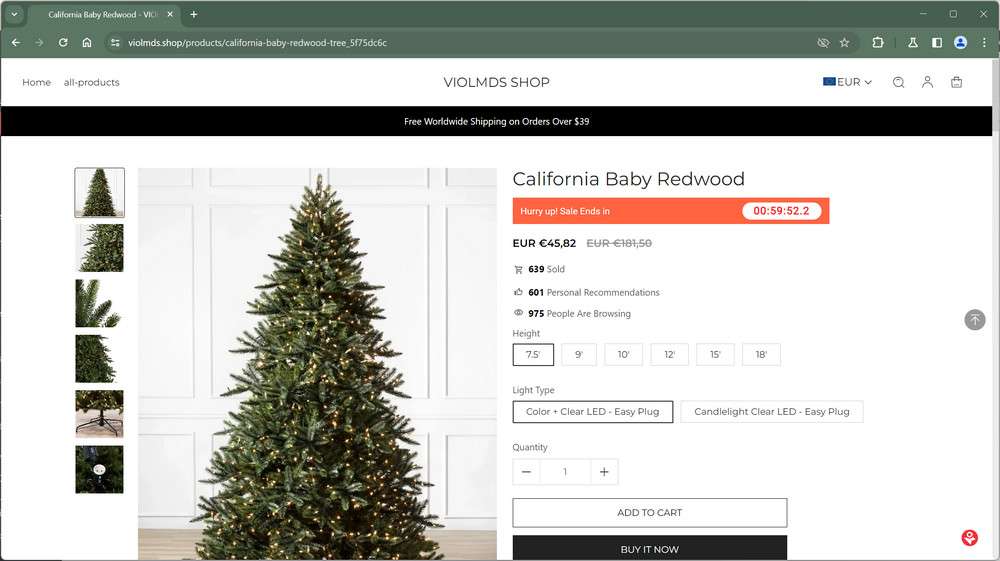This image captures a detailed screenshot of the website "VEIOLMDS SHOP". At the top of the page, there is a navigation bar with several elements. On the left side, there is a "Home" button, followed by an "All Products" button. Centrally placed is the website's name, "VEIOLMDS SHOP," in bold, capital letters. Towards the right side of the navigation bar, an option for the European version of the site is presented, offering translated categories. Additionally, there are three icons: a magnifying glass for search, a person icon presumably for user accounts, and a cart icon for shopping.

Below the navigation bar is a prominent section featuring the "California Baby Redwood" artificial Christmas tree. On the left side of this section, six thumbnail images show different views of the tree, allowing users to select and view more details. To the right, a larger, full-size image of the selected thumbnail is displayed.

Adjacent to the images, the product details are clearly outlined. The title "California Baby Redwood" is prominently displayed. Beneath it, a countdown timer is shown, followed by the product's price listed in euros. Additional information includes the number of units sold, the number of recommendations, and the current number of people viewing the product.

Options for customizing the tree are listed further down. Users can choose from various heights: 7.5 feet, 9 feet, 10 feet, 12 feet, 15 feet, and 18 feet. There are also options for different light types: a color button and a candlelight button. Below these options, there is a quantity selector and an "Add to Cart" button for completing the purchase.